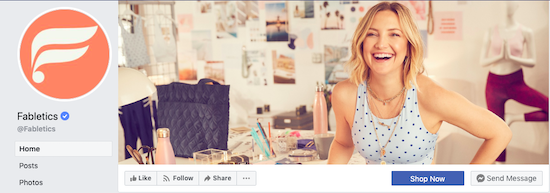Kate Hudson, the renowned actress and founder of the activewear brand Fabletics, is depicted here in a promotional image for the Fabletics website. Seated at a desk, she beams a warm smile while showcasing her casual yet chic style in a polka dot tank top paired with a gold necklace. Behind her, a mannequin strikes a yoga pose with hands pressed together, dressed in a top and maroon stretchy pants, representing the brand's stylish and functional apparel.

The backdrop features a collection of posters, flyers, and prototypes, hinting at the creative process and dynamic environment of the Fabletics workspace. On the left side of the image, the prominent white "F" logo encircled in orange signifies the Fabletics brand. Underneath, the word "Fabletics" is displayed alongside a check mark, reminiscent of Twitter’s verified badge, further indicating the brand's authenticity and presence on social media.

The website interface shown includes a navigation column on the left, highlighted and bolded on the "Home" section, indicating the current page. Below the smiling image of Kate, a blue "Shop Now" button invites users to explore the merchandise, flanked by a gray "Send Message" button. There are also interactive options to like, follow, or share the content, with additional options accessible via a three-dot menu.

This image not only highlights Kate Hudson's involvement and personal connection to Fabletics but also emphasizes the brand's dedication to delivering high-quality, stylish athletic wear.